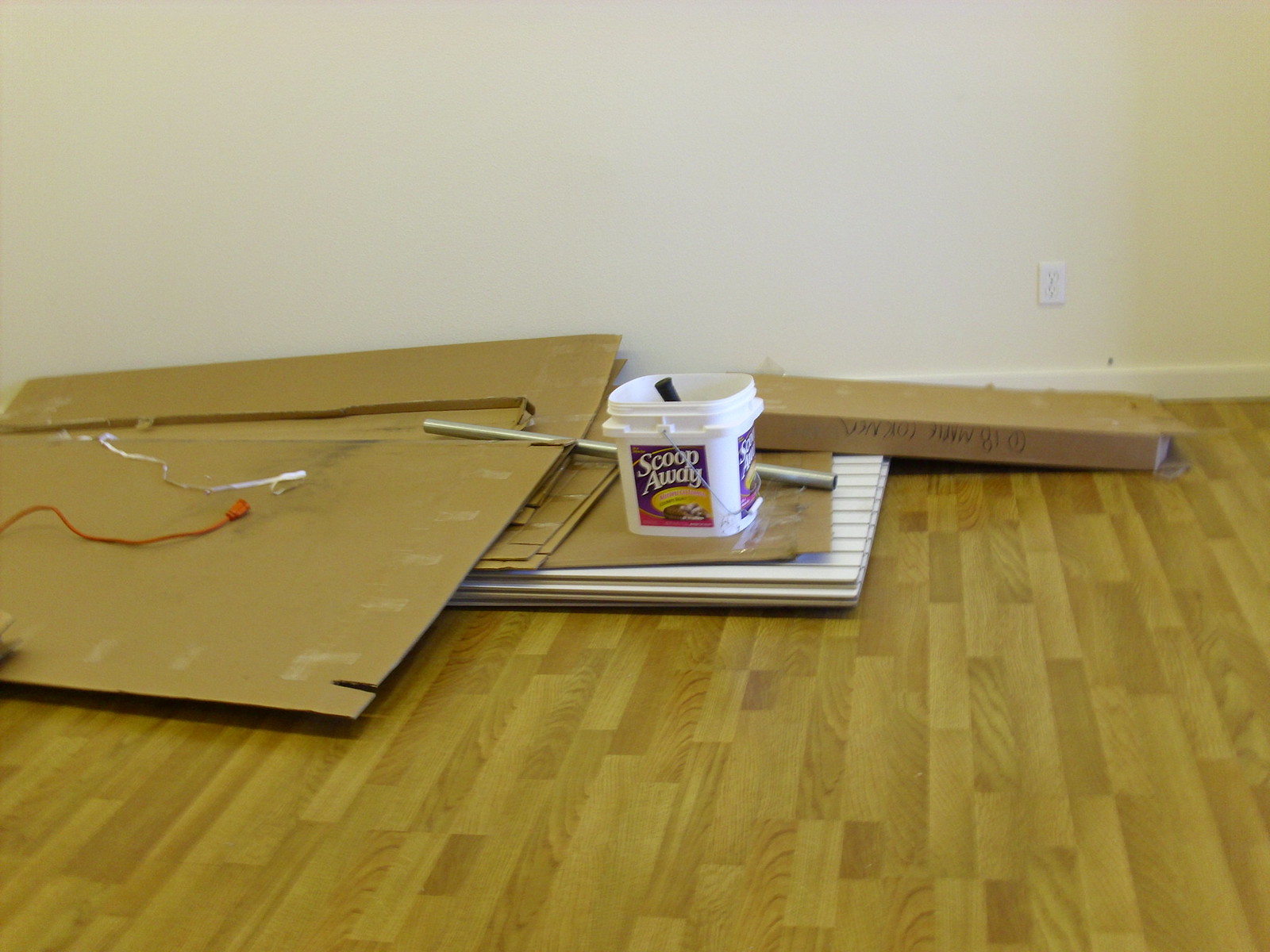The room in the house features white, slightly textured walls with an electric outlet positioned on the lower right side. The floor is composed of hardwood, with a light-colored finish. In one corner, there is a pile containing numerous flattened cardboard boxes stacked on a white-striped base. Among the boxes, an orange extension cord extends to the left, while a piece of tape is partially peeled from one of the boxes. Resting in the center of the pile is a hollow metal rod, approximately two feet long and wide enough to fit comfortably in a hand. Behind the flattened boxes, an un-collapsed box marked with some lettering, including "118", sits on the right. Atop this arrangement is another cardboard box, which is crowned with a white pail used for cat litter, labeled "Scoop Away". Additionally, a black handle protrudes from the top of this pail.